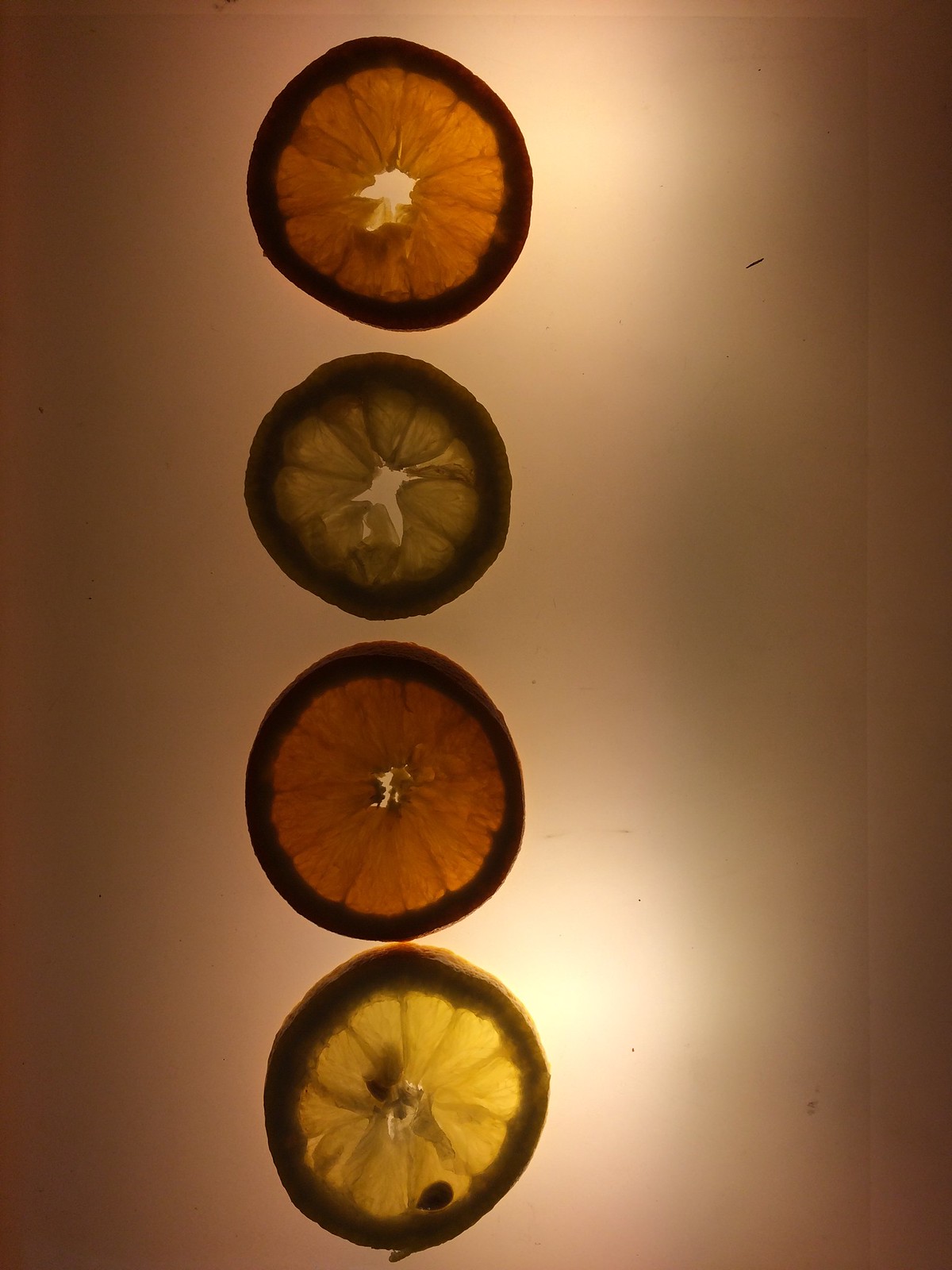This photograph captures a downward view of a table with a neat vertical row of four dried citrus fruit slices. The background transitions from dark black with pink edges to a lighter pink towards the center. Starting from the top, the first slice appears to be an orange with a dark rind and a paper-thin, dark orange interior, featuring a central hole that exposes the table beneath. The second slice looks like a lime, distinguished by its dark green rind and light green interior, also with a central hole. The third slice resembles another dried orange, with similar dark outer edges and orangish, almost transparent middle. The fourth and bottommost slice is likely a lemon, displaying a dark green rind, a slightly greenish interior and containing one visible seed at the bottom. The arrangement of the slices is slightly left of center on the table, emphasizing their delicate and dried nature.